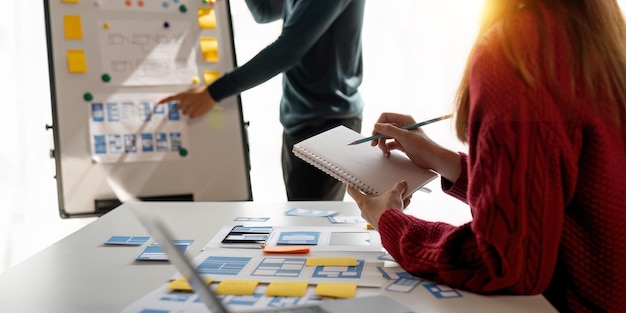In this detailed image, two people are engaged in what appears to be a meeting. The woman, wearing a red cable-knit sweater, has long hair that is a mix of brown and blonde. She is seated at a white table covered with various pieces of paper featuring blue tables and graphs, alongside yellow, white, and orange sticky notes. She holds a blue-colored pencil poised over a spiral-bound notebook, looking attentive as she appears to take notes. In front of her sits an open laptop and more scattered yellow sticky notes and blue-and-white diagrams. 

Opposite her stands a man clad in a green light sweater. His left hand points to a piece of paper with blue and white squares on the table, as he presents information. Behind him is a white board adorned with several yellow sticky notes arranged on both sides - three on the right and two on the left. The central section of the board displays a white paper with interconnected black and white squares held up by magnets in yellow, purple, and green. Below it, another white paper with blue squares is secured by two green magnets at the corners. Both individuals are focused and engaged, immersed in what appears to be a thorough discussion or presentation.